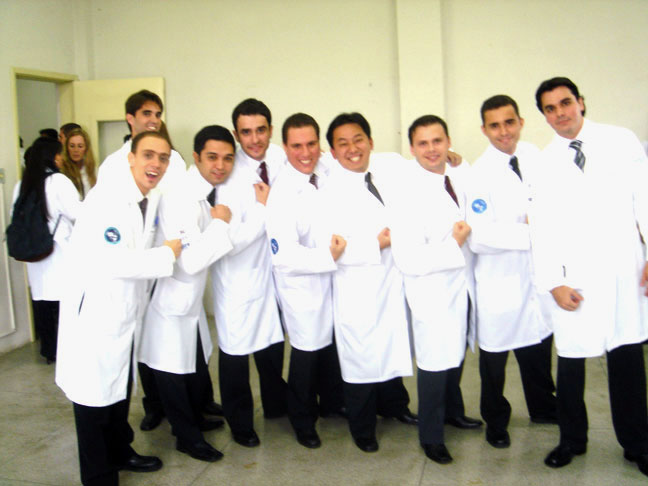In this photograph, nine young men, likely in their 20s to 30s, stand side by side facing the camera, exuding a sense of camaraderie with their right arms bent and fists raised in a confident "we're cool" gesture. Each man is dressed uniformly in a long, white lab coat that almost glows with brightness, complemented by dark-colored ties, black pants, and black shoes. Among the group, there are two Asian men—one in the center and another slightly to the left—while the rest of the men vary in ethnicity, including Hispanic, white, and possibly Italian or Greek.

The men are all smiling, creating a friendly and approachable ambiance. On the upper right arm of a few lab coats, a round blue patch, possibly indicating their affiliation with an organization like NASA, suggests they might be scientists or engineers. The background showcases a large room with a beige floor made of large tiles and off-white to yellowish walls. On the left side of the image, an open, muted yellow door reveals two women—one with dark hair and the other blonde—deep in conversation, while another person in a lab coat with a large black backpack stands in the doorway. The overall setting hints at a professional or institutional environment, adding depth to the image's narrative.